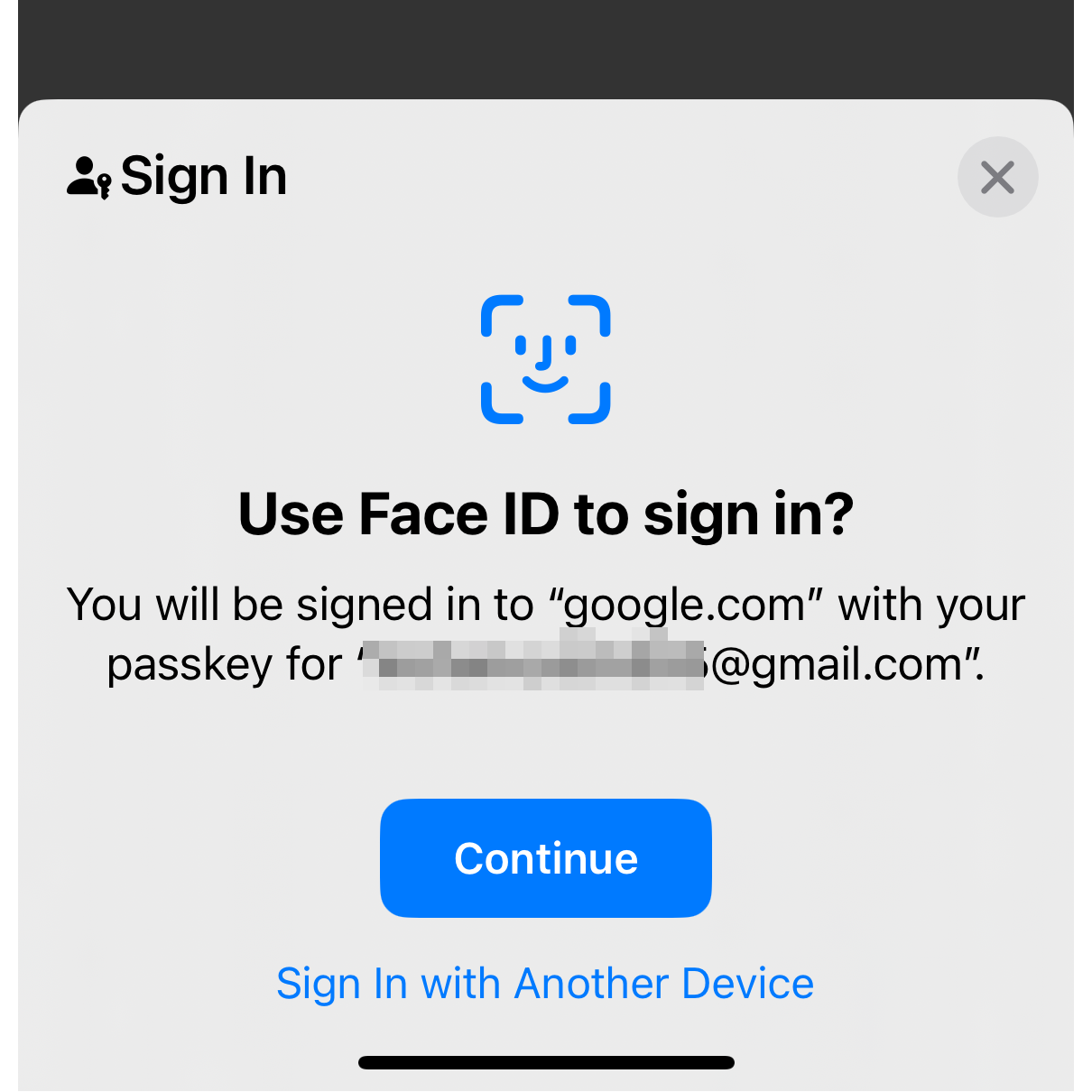In this image, there is a screenshot of a mobile phone screen. At the top, a black band is visible, possibly part of the phone's interface. Below it, a pop-up window appears, featuring a light grey or white background with light green accents. 

At the top of the pop-up, the word "Sign In" is written in black ink, with an "X" icon for canceling the prompt on the right side. The middle section of the pop-up includes a blue ink drawing of an emoji-like face, accompanied by the text "Use Face ID to sign in" in black ink. 

Further down, a notice in black ink explains, "You will be signed in to google.com with your passkey for..." followed by an email address. For privacy, most of the email has been obscured, displaying only "****@gmail.com" with the obscured part appearing bled out in black ink. 

At the bottom of the pop-up, there is a blue box containing the word "Continue" in white ink. Below this box, the text "Sign in with another device" is written in blue ink.